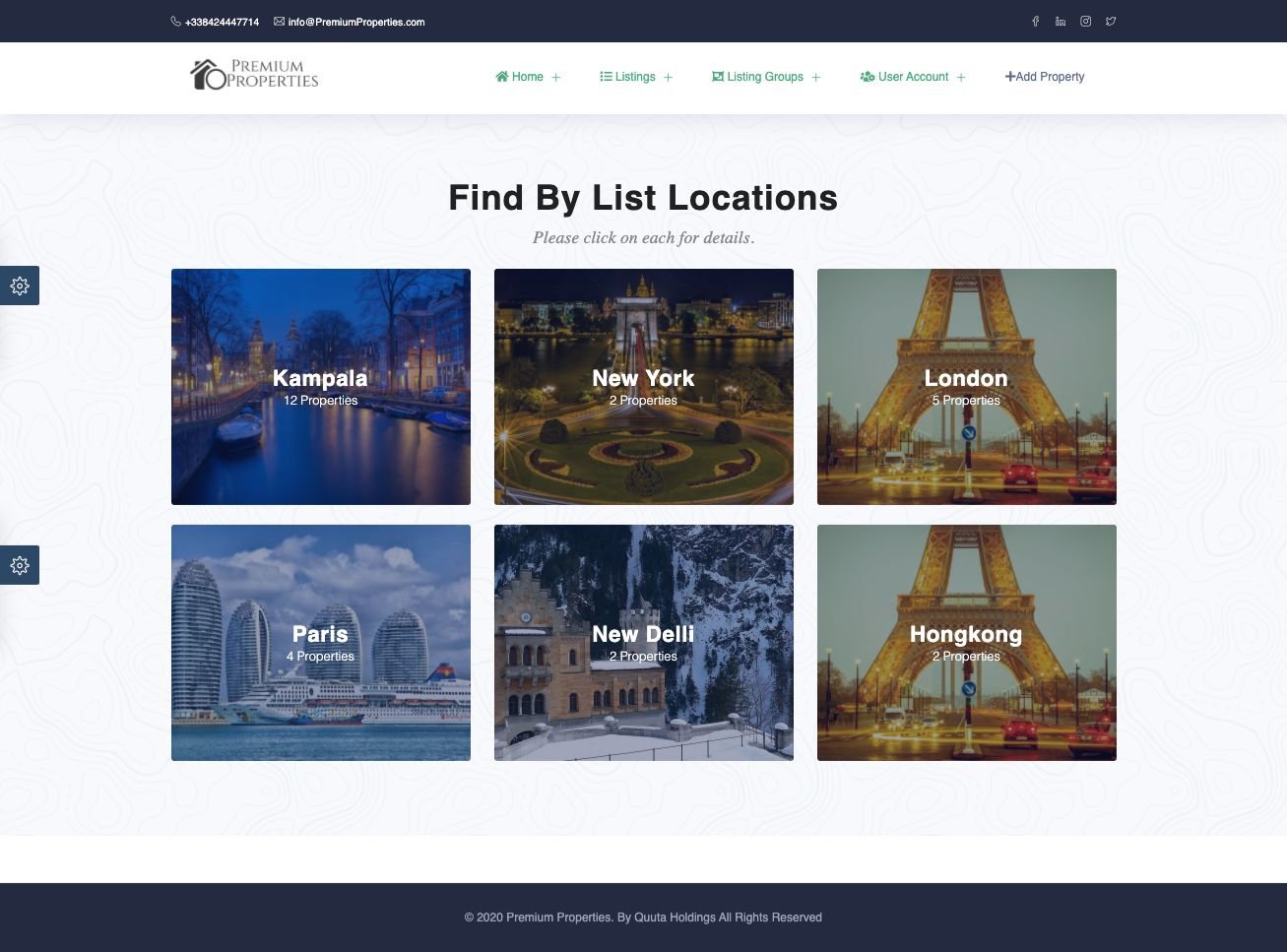Screenshot of the Premium Properties website displaying international real estate listings. The website's navigation bar features five tabs at the top: Home, Listings, Listing Groups, User Account, and Add a Property. Below these tabs, six images are arranged in two rows under the section "Find by List Locations," showcasing various property locations.

In the first row:
- Kampala: **12 properties** are listed, accompanied by an image representing Kampala's cityscape.
- New York: **2 properties** are listed, with a relevant image of the city.
- London: **5 properties** are listed; however, the background mistakenly features the Eiffel Tower, which is actually located in Paris.

In the second row:
- Paris: **4 properties** are listed, but the background image mistakenly depicts a scene resembling a Middle Eastern country with cruise ships.
- New Delhi: **2 properties** are listed, but the associated image inaccurately shows a snowy, mountainous landscape resembling a European castle.
- Hong Kong: **2 properties** are listed, erroneously using another image of the Eiffel Tower.

The inconsistencies in the background images highlight a need for more accurate visual representation of the listed locations.